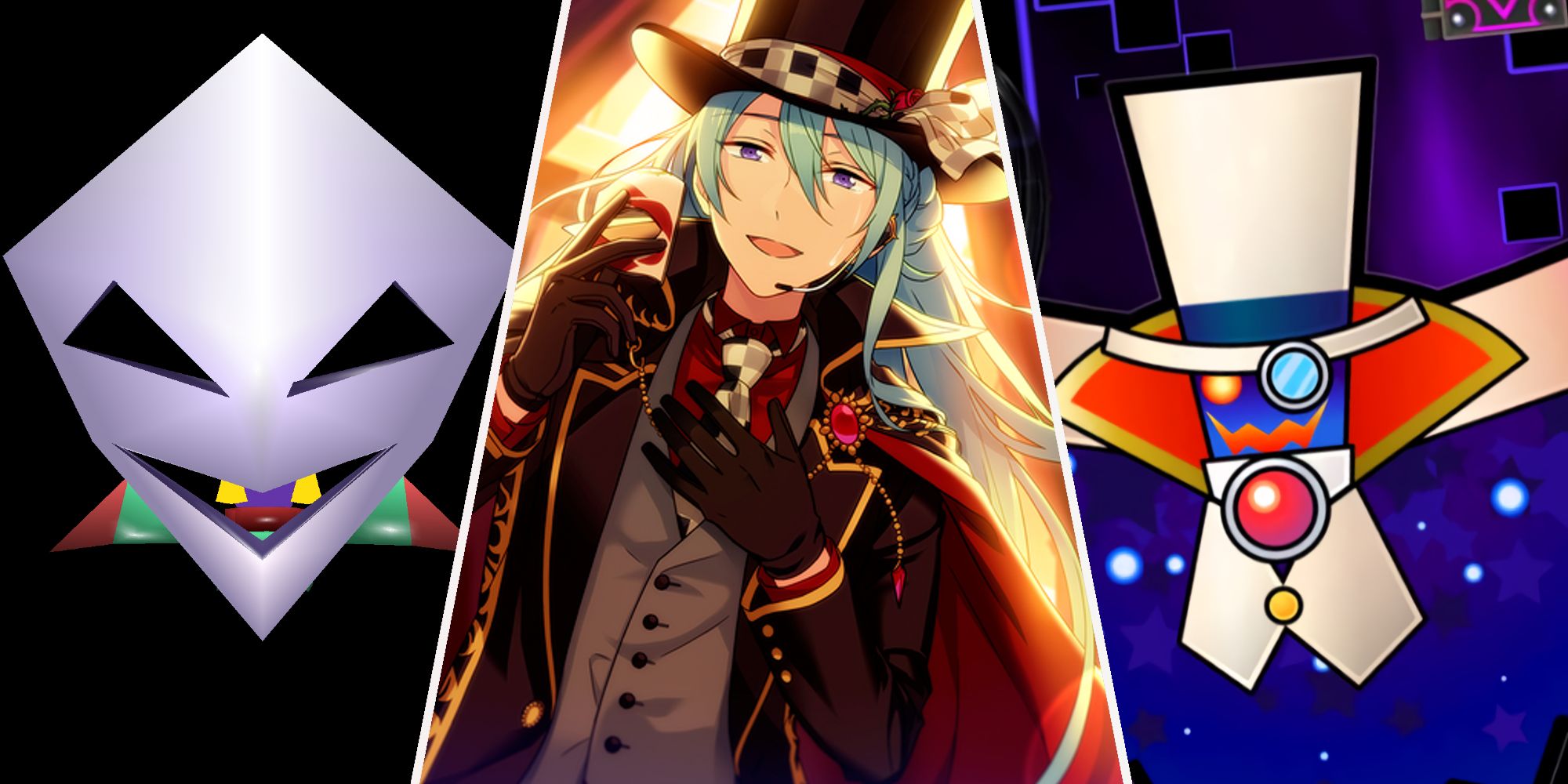The horizontally laid image is divided into three distinct sections, each showcasing a unique style. The center section features a manga-style illustration of an androgynous youth, possibly a girl, adorned in a striking outfit reminiscent of a conductor's jacket—not unlike something Michael Jackson might have worn. She wears a brown top hat and a headpiece with a visible mouthpiece. Her ensemble includes a gray vest, a maroon shirt, and a checked necktie in shades of white, black, and tan. An emerald brooch or cloak clip decorates her left shoulder, and she dons brown gloves, holding an indistinguishable object in her right hand. She has light skin, green hair, and blue eyes, and is positioned looking straight ahead.

Flanking this central image are two cartoon-style pictures. On the left is a simple 3D-generated image of a smiling jack-o-lantern-like mask in gray, featuring two yellow teeth, a tongue, and a neck and shoulder area that appears airbrushed in green and red hues. On the right is a color illustration of a caricature, depicting a robot or man with a top hat and monocle, somewhat reminiscent of Mr. Peanut. This figure's neck area is represented by a domed red button or sensor, set against a cosmic blue background adorned with glowing white dots.